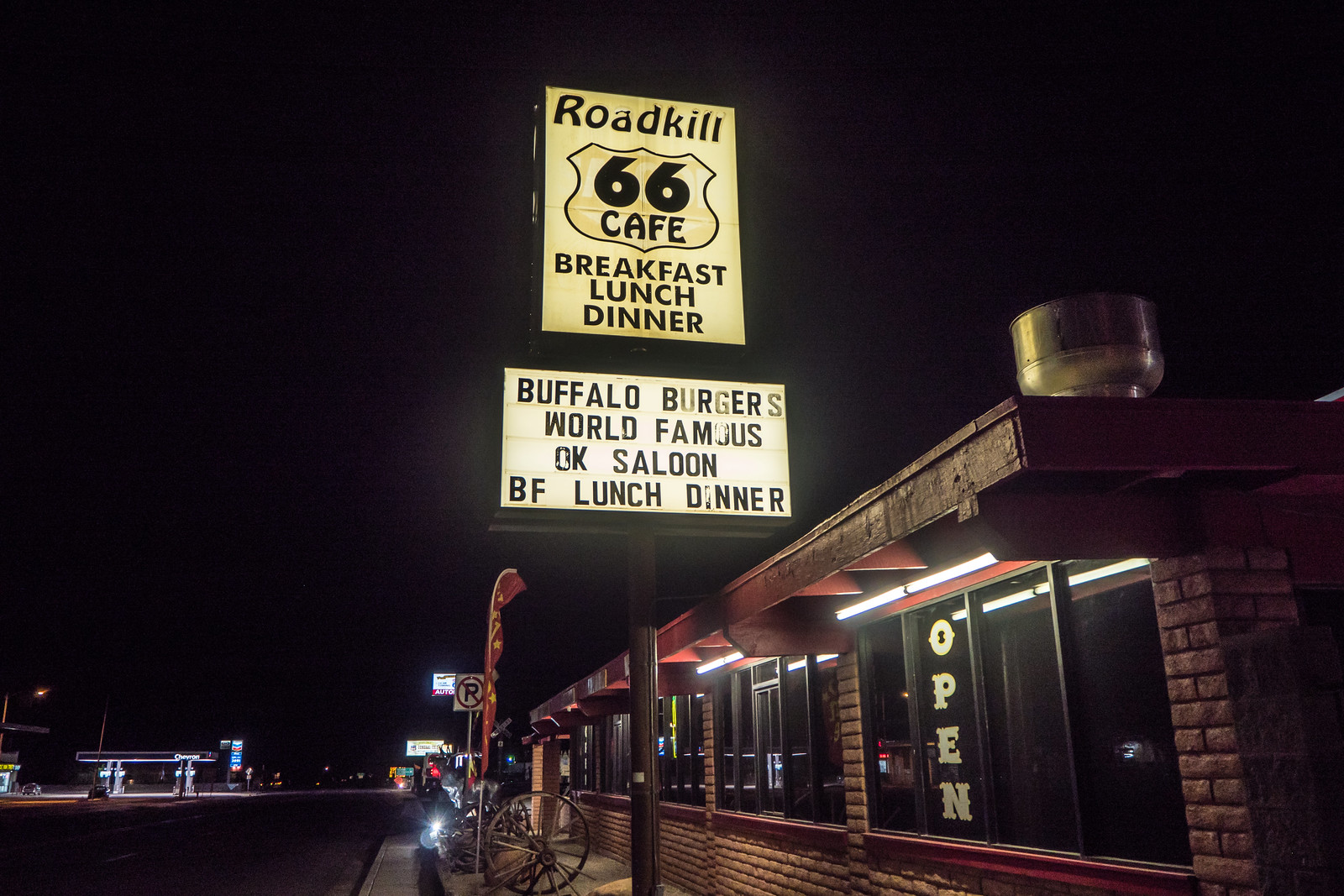The photograph, taken at night, features a horizontally aligned rectangular view with a pitch-black sky occupying the upper half as a backdrop. Captured at a slightly upward angle, the image centers on a lighted sign outside a restaurant named "Roadkill 66 Cafe" which offers Breakfast, Lunch, and Dinner. Directly beneath this main sign, another illuminated sign announces "Buffalo Burgers - World Famous - OK Saloon" followed by "BF Lunch Dinner".

The scene includes a single-story brick building constructed of brownstone on the right side, distinguished by several rectangular, black windows. One of these windows displays the word "Open" in vertical, white letters. The building also features fluorescent lights on the ceiling of its covered exterior area, enhancing visibility.

A large wheel that resembles one from a carriage is visible but no carriage is present. In the left background, the street appears empty with no cars, and across the street, a Chevron gas station sign is discernible along with the familiar Chevron colors and gas prices.